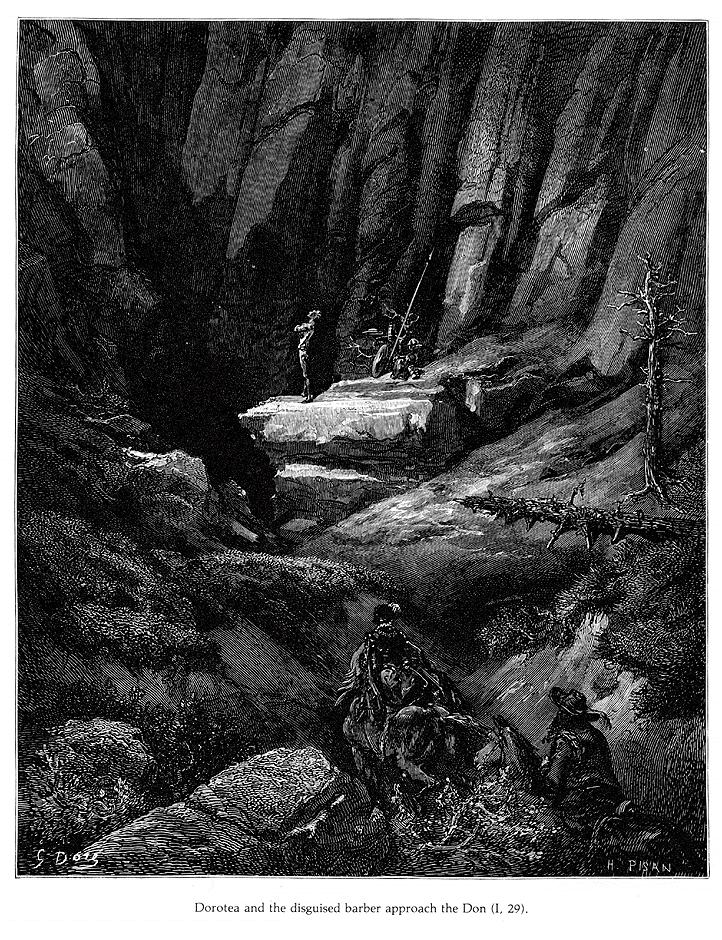The artwork, possibly created using etching or stippling techniques, is a detailed black and white piece titled "Dorotea and the Disguised Barber Approach the Dawn, 1,29," and signed by H.PISAN. The scene is characterized by stark contrasts of heavy dark tones and bright white spaces, lending depth and drama to the composition. Highly detailed rock formations dominate the middle ground, where a light-colored silhouette of a person with their arms crossed gazes upwards, positioned on an illuminated rock formation. Adjacent to this figure, leafless trees - one fallen and another still rooted - add to the barren landscape. 

In the foreground, there is a complex interaction involving a person seemingly grabbing onto another figure or object while lying down on what could be a grassy patch. Directly opposite, another individual on horseback, donned with a hat and beard, confronts the scene. Additionally, the bottom-right corner of the image features two horse-riding travelers navigating the rocky terrain towards the central silhouetted figure, enhancing the sense of journey and discovery within the piece. The initials "H.PISAN" are inscribed in the lower portion, solidifying the artist's identity.